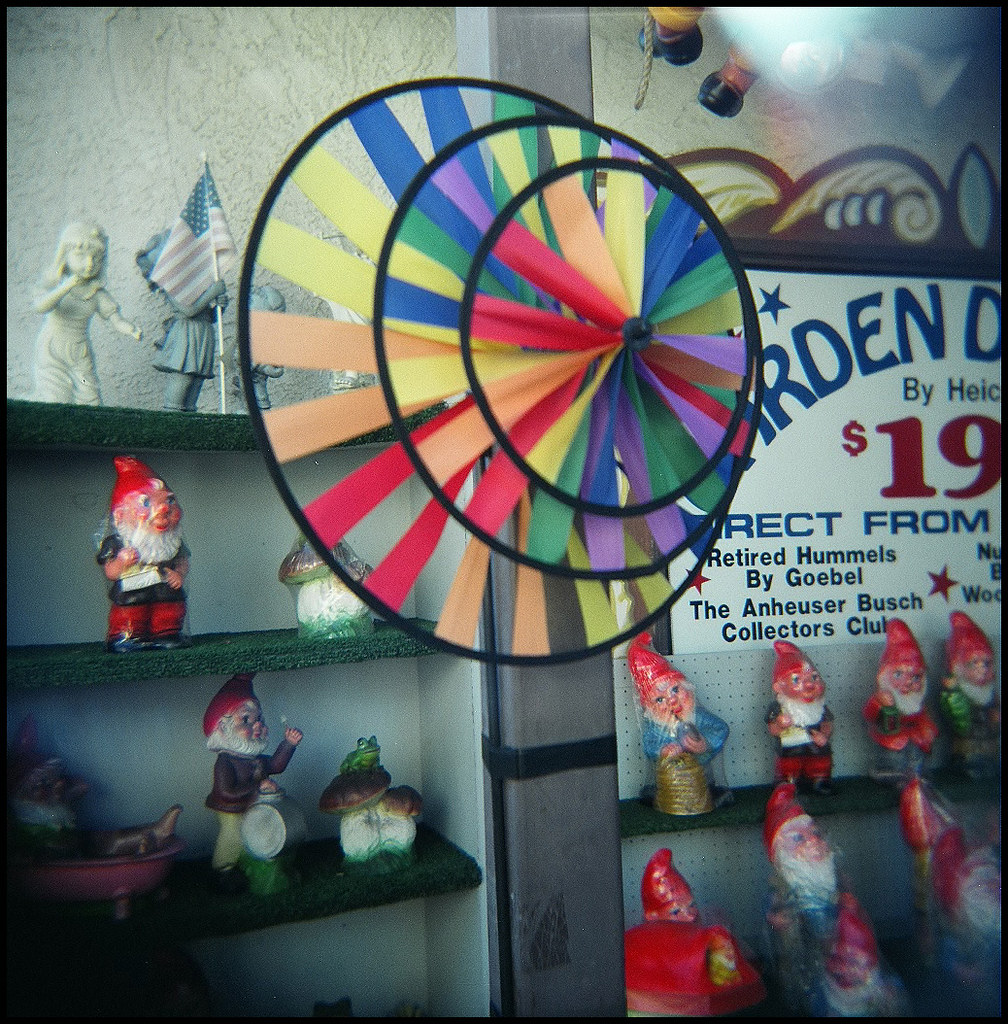The image depicts an indoor store scene featuring a cabinet with multiple green shelves, each adorned with various whimsical gnome statuettes and other garden-themed decorations. On the top shelf, there's a gnome holding an American flag alongside a little statue of a girl. Below it, there's a fanciful mushroom with a purple top and a white and green bottom, next to another gnome. The next shelf down showcases a gnome relaxing in a small pink bathtub and a different mushroom with a frog perched on it. Another gnome appears to be playing a drum. Dominating the foreground of the image is a vibrant, colorful wind spinner, likely intended for garden use. A partially visible white sign suggests that these items are retired Hummels by Goebel, associated with the Anheuser-Busch Collectors Club. The arrangement is somewhat scattered, with a variety of colors including white, green, brown, tan, red, blue, pink, orange, and yellow, adding to the eclectic and playful atmosphere of the display.